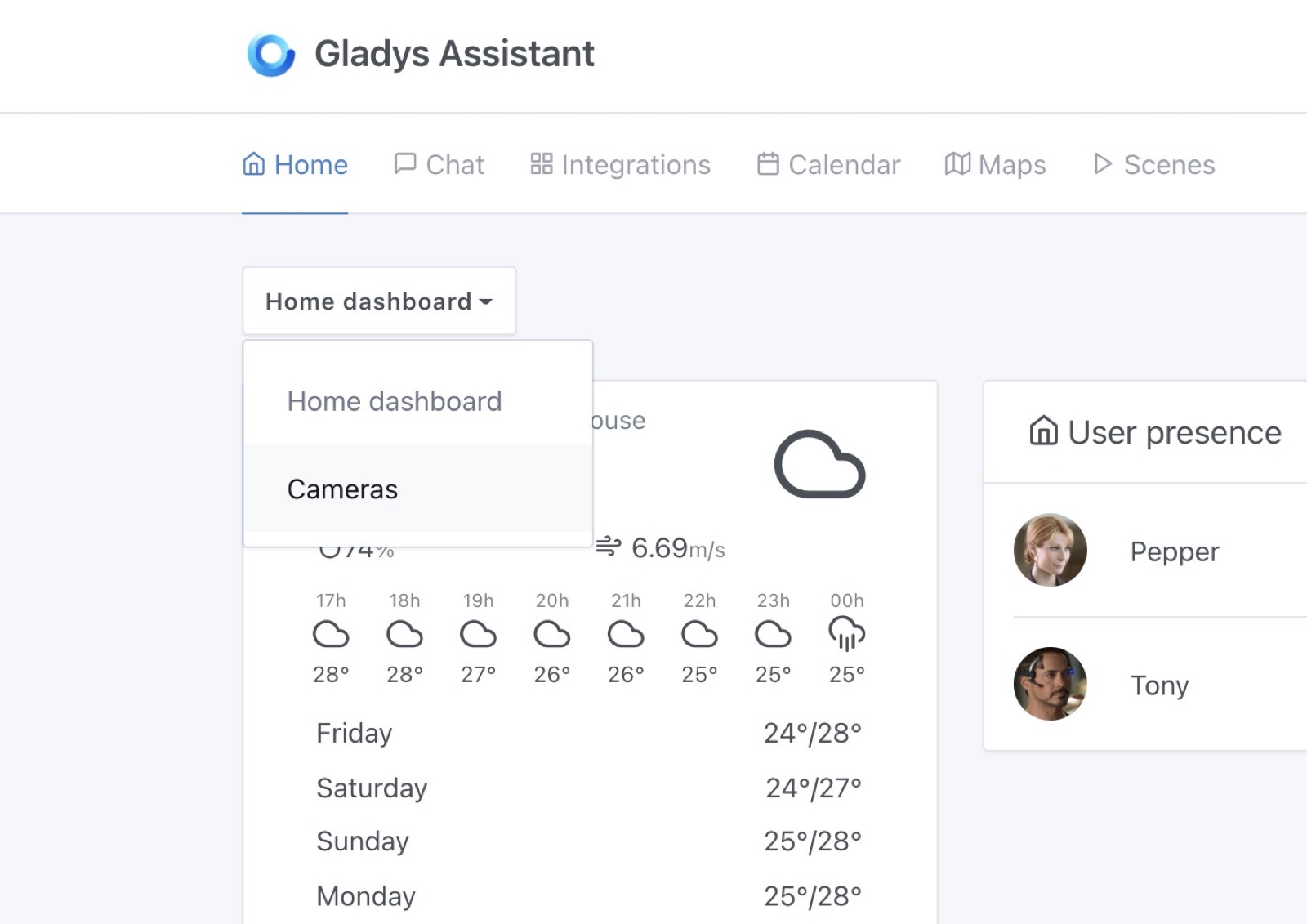This is an image that appears to be a screenshot from a computer, showcasing the interface of a digital assistant application named "Gladys Assistant." In the upper left corner, there is a blue circle followed by the name "Gladys Assistant." Below that, there's a navigation bar where different categories can be selected. Currently, the "Home" category is selected, indicated by its blue color and underlined home icon. Other categories listed, in gray, include Chat, Integrations, Calendar, Maps, and Scenes.

Underneath the navigation bar, the text "Home Dashboard" is visible. An arrow has been clicked, revealing a submenu that reads "Home Dashboard, Cameras," with "Cameras" highlighted. The interface is superimposed over another image. 

Within this lower image, there's a square box displaying the weather forecast with icons and temperatures for various times of the day, including 28 degrees and 26 degrees. The forecast for Friday through Monday is listed vertically. 

To the right of the weather information, there’s another small box labeled "User Presence," featuring the icon of a house. Below this, two circular profile pictures are shown. The top image is of a woman, labeled "Pepper," and the second of a man, labeled "Tony." Both individuals appear to be Caucasian.